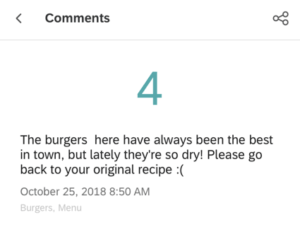A detailed caption for the given description could be:

---

The snippet features a review segment from a restaurant review web page. The user has rated the restaurant a "4" (in green, suggesting it's likely 4 out of 5) and the headline "Comments" is prominently displayed. Below the rating, the reviewer expresses their disappointment with the restaurant’s current burger quality: "The burgers here have always been the best in town, but lately they're so dry. Please go back to your original recipe :(" The review is timestamped "October 25, 2018 at 8:50 a.m." The faint text beneath, difficult to decipher, starts with "Burgers" and includes another word beginning with "M". The entire segment is styled in a grayish font, making it less readable. The green rating number resembles a popular color seen often on modern cars. A left arrow next to "Comments" suggests navigation to a previous screen, while three interconnected dots on the right likely offer additional menu options.